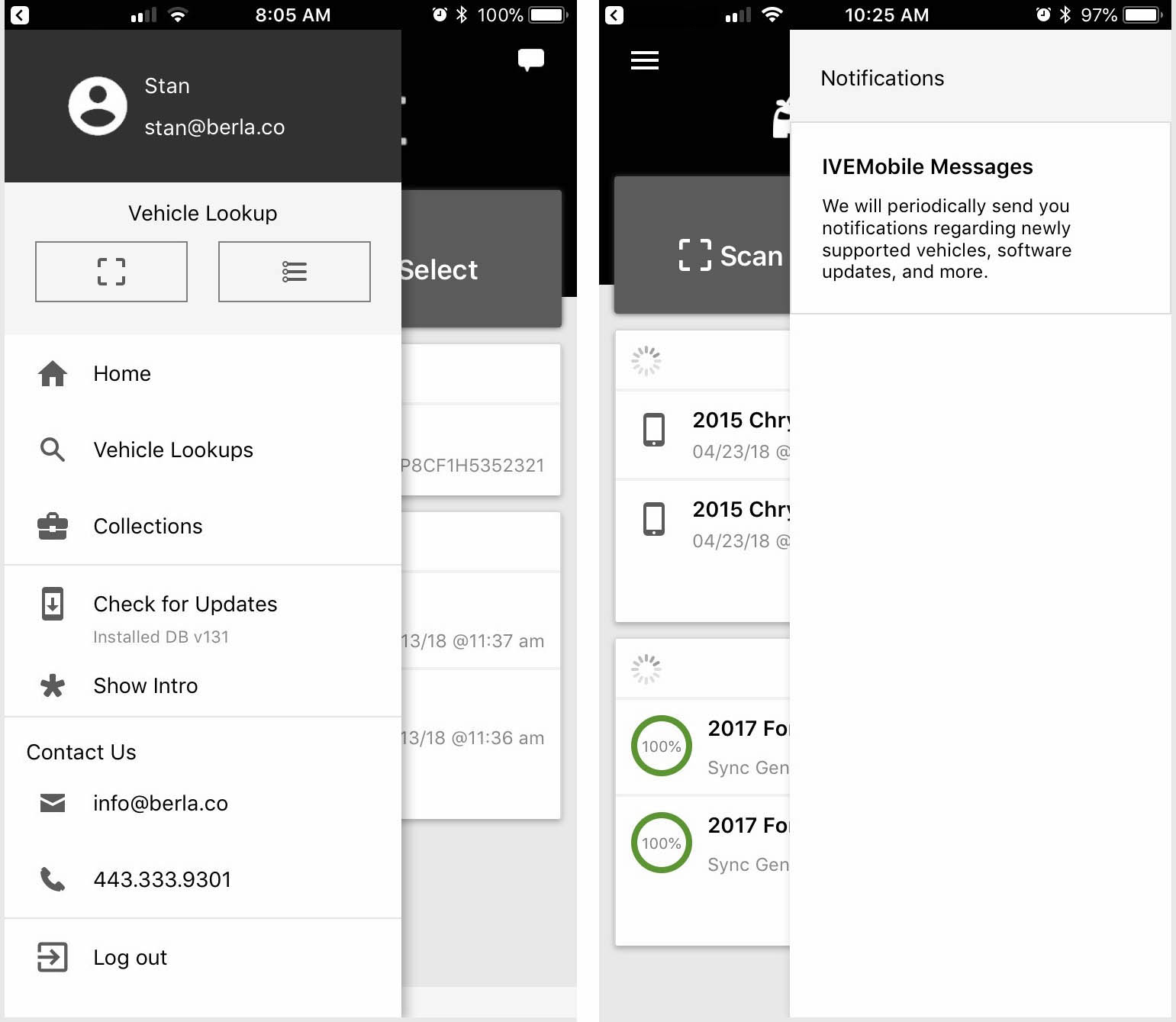Here are two detailed descriptions for the respective screenshots:

**Screenshot 1 (8:05 a.m., 100% Battery):**
The first screenshot displays a webpage from Burla.co taken at 8:05 a.m., with the device showing a fully charged battery at 100%. At the top left corner of the interface, there is a clear label "Stand" followed by "stand at burla.co." Key navigation elements include the "Vehicle Lookup" option, a square icon, and a hamburger menu symbolized by three circles aligned vertically. The menu, positioned at the left end of the page, expands to show options such as "Home," "Vehicle Lookups," "Collections," "Check for Updates," "Show Intro," "Contact Us," and "Logout." Specific contact details provided are an email address (info@burla.co) and a phone number (443-333-9301). On the right side, there is a notifications section titled "IVE Mobile Messages," with the letters "I," "V," "E," and "M" prominently capitalized. This section informs users about periodic notifications regarding newly supported vehicles, software updates, and more.

**Screenshot 2 (10:25 a.m., 97% Battery):**
The second screenshot, captured at 10:25 a.m., shows a slightly depleted battery at 97%. Similar to the first image, the page belongs to Burla.co but without any notable changes in content or layout. The same menu options and contact details are present as in the first screenshot, with "Stand" at the top and a focus on "Vehicle Lookup." The "IVE Mobile Messages" notification section remains prominently on the right side, continuing to inform users about receiving updates and relevant notifications.